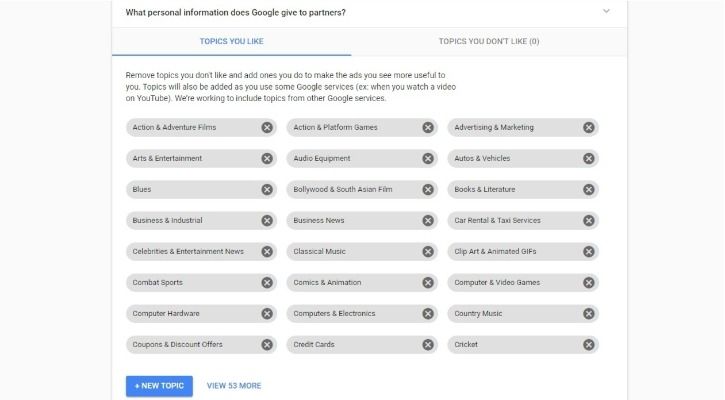This detailed description refers to an informational page about managing personal information shared with Google and its partners. The page discusses the customization of topics for targeted advertising purposes. Here is a cleaned-up and more descriptive caption for this image:

"An informational Google page explaining how to manage personal information shared with partners for enhanced ad personalization. The header poses the question, 'What personal information does Google give to partners?' Two sections are indicated: 'Topics you like' and 'Topics you don't like.' Currently, only 'Topics you like' is selected, highlighted in blue text with a blue underline. Instructions suggest removing or adding topics to tailor the ads you see, noting that topics will also accumulate based on your activity across various Google services, such as watching YouTube videos.

Displayed topics are organized in gray capsule-shaped tags, each featuring a close-button (cross) on the right for easy removal. Some examples of topics include Action Adventure Films, Arts and Entertainment, Blues, Business and Industrial, Celebrities and Entertainment News, and many more, collectively spanning a broad array of interests from business to entertainment to sports.

At the bottom left of the page are two interactive elements: a blue button labeled 'Add a new topic' and a blue text link, devoid of an outline, reading 'View 53 more,' providing users with further customization options."